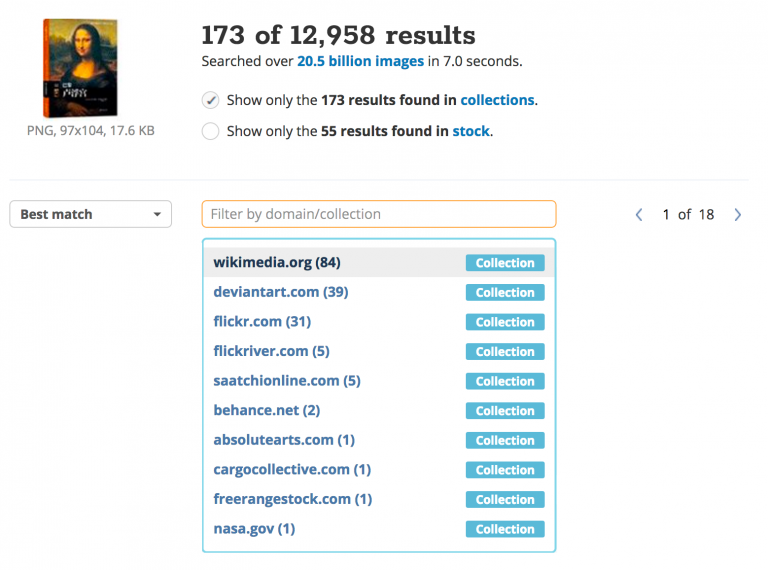**Detailed Caption**:
This color image is a screenshot of an image search result interface. The top section of the interface features a predominantly white background with black and blue text. Prominently displayed at the top is a thumbnail of Leonardo da Vinci's iconic painting, the Mona Lisa. Accompanying the thumbnail is a label indicating the image's dimensions (97 by 104 pixels) and its file size (17.6 KB). 

Further details at the top reveal that the search yielded 173 results out of a total of 12,958, having scanned over 20.5 billion images in just 7 seconds. The interface offers options in the form of radio buttons to filter the results. The selected option is "show only the 173 results found in collections," while the alternate, unselected option is "show only the 55 results found in stock."

Below these filtering options, the results page is displayed. On the left, there is a label indicating "best match," and on the right, navigation controls with page numbers and forward/backward arrows indicate that this is page 1 of 18. There is also a dropdown menu with faint gray placeholder text that reads "filter by domain collection."

The search results are organized into a list of image collections, with each collection specified by source names such as Wikimedia, DeviantArt, Flickr, Flickr River, Saatchi Online (spelled S-A-A-T-C-H-I Online), and NASA.gov, among others. Next to each collection name, the number of Mona Lisa images available within that collection is listed, for instance, NASA.gov has 1 image, and Wikimedia has 84 images.